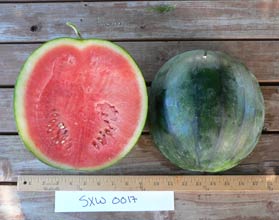The image features a perfectly round watermelon, darker green with striations on a lighter green background. The watermelon is neatly cut in half from stem to base. The left half, with its coral red flesh and a scattering of mostly white seeds, is displayed cut-side up. The right half, showing the green rind, is displayed cut-side down. The cut reveals a very pale green, almost white inner rind. Both halves rest on an unfinished wooden surface, likely part of a display, possibly for a farm or gardening show. A ruler lies beneath them, measuring approximately 16-17 inches across, with a strip of white paper labeled "SXW0017" at the bottom. The image is taken from an overhead perspective, highlighting the detailed arrangement.